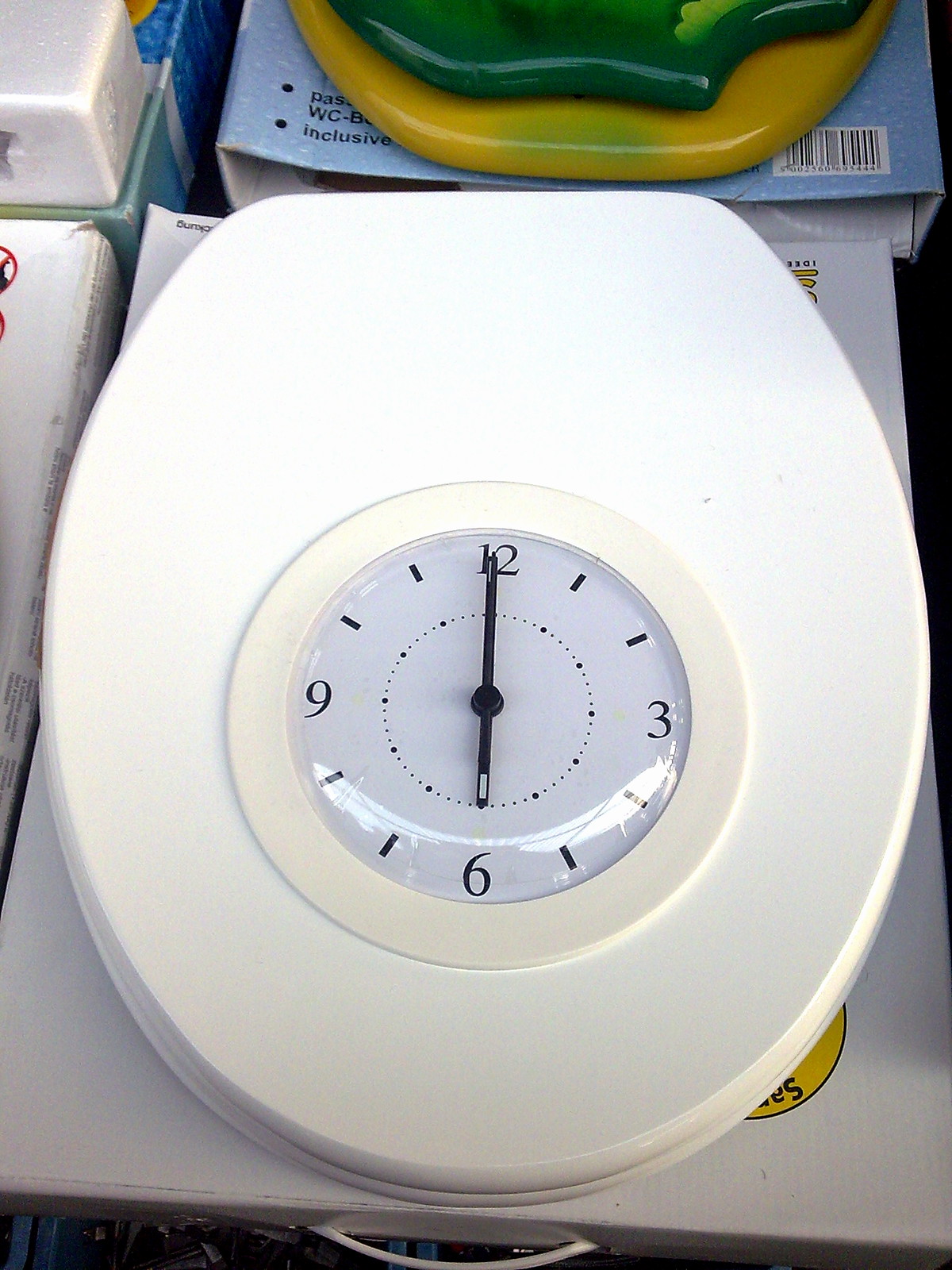The image showcases an unconventional setup where a toilet seat is positioned atop a white case. Extending from the bottom middle of the case is a handle. At the center of the top part of the toilet seat, there is an analog clock with a white face displaying black numerals—specifically 12, 3, 6, and 9. The other hours are marked by dashes. The clock shows the time as 6 p.m. and features a white frame surrounding the clock face, which reflects some light. Behind the toilet seat, a yellow plastic item is placed, resting on a light blue box situated at the very top middle of the photo. In the upper left corner, several cardboard boxes are partially visible, adding to the cluttered scene.